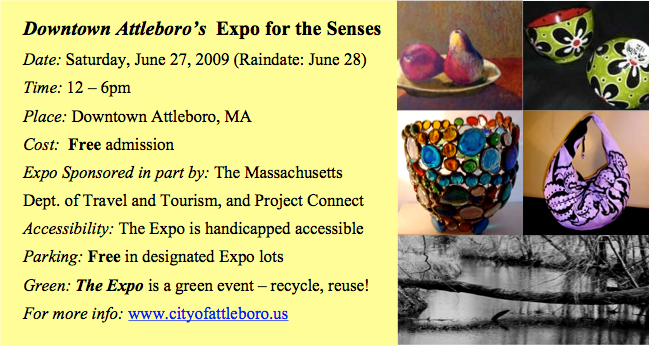The image is a vibrant advertisement for the "Downtown Attleboro's Expo for the Senses," scheduled for Saturday, June 27, 2009, from 12 to 6 p.m., with a rain date on June 28th. The event will be held in downtown Attleboro, Massachusetts, and offers free admission to all attendees. Sponsored in part by the Massachusetts Department of Travel and Tourism and Project Connect, the Expo is handicapped accessible with designated free parking. It promotes sustainability with a green initiative encouraging recycling and reuse. 

The advertisement is divided into two sections: a larger text block on the left and an array of colorful images on the right. The left section features a light yellow background with detailed black text outlining the event specifics, including the website for more information, www.cityofattleboro.us.

The right section showcases five pieces of art: 
1. A painted picture of two pears on a glass plate, vibrant with pink hues.
2. A pair of green bowls adorned with black flowers, featuring white centers and red interiors.
3. An intricate blown glass art piece with shades of yellow, blue, green, and red.
4. An ambiguous item, possibly a vase or bag, illustrated in black and pale purple.
5. A horizontal black and white photograph of a tree trunk forming a small bridge over water, providing a serene natural element to the collection.

The overall design is professional and colorful, effectively conveying the artistic and inclusive spirit of the Expo.